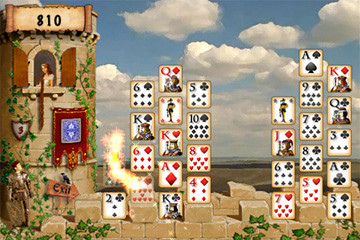In this detailed screenshot from a video game, we see a card game interface set against a medieval-themed background. The right-hand side of the image showcases a serene blue sky dotted with puffy white clouds that become densely clustered lower down. Dominating the left side is a tall, tan brick tower adorned with prolific green vines. At the top of the tower, a scroll-like banner displays $10. An arched window with brown shutters houses a woman who appears to be Rapunzel, characterized by her long, flowing brunette hair and white dress, as she gazes outward. Below her, at the base of the tower, a man—presumably a prince with dark clothing and brown hair—looks up at her. Nearby, an 'EXIT' sign with a bird perched on it points downward. In front of this fairy-tale backdrop, the card game features seven vertical rows of cards. Prominent among the displayed cards are the 10 of diamonds, 8 of hearts, queen of diamonds, six of spades, king of spades, six of diamonds, two of clubs, king of clubs, ace of diamonds, king of hearts, five of clubs, ten of spades, four of diamonds, and a notably burning card on the left-hand side.